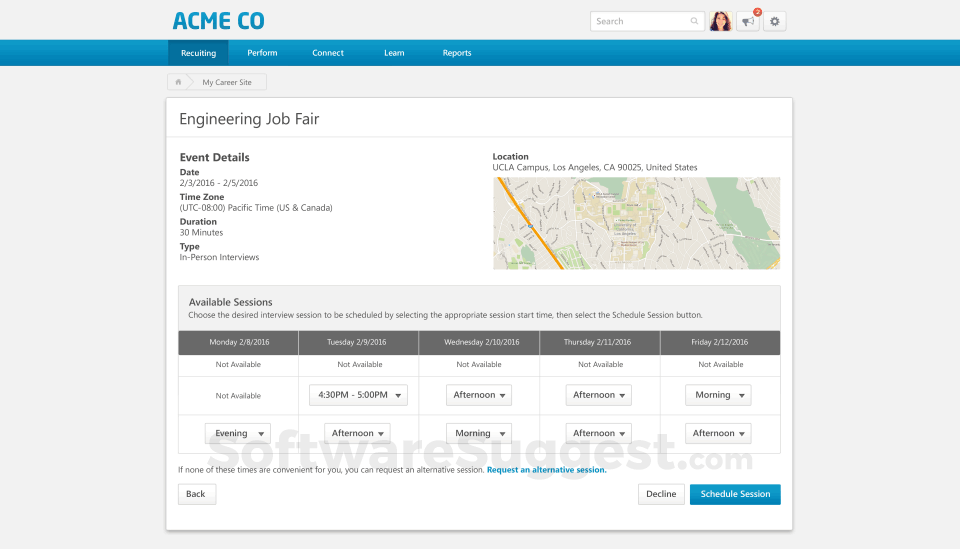The webpage displayed belongs to Acme Co., a company known as Acme Space COS. In the top-right corner of the page, there is a search bar, which suggests that a young white woman is currently signed in. She has two unread messages denoted by a small icon, alongside a gear icon that presumably represents the settings menu.

Beneath this top section, there's a blue navigation bar featuring several tabs: "Recruiting," "Perform," "Connect," "Learn," and "Reports." The active tab is "Recruiting," which leads to information about an upcoming event titled "Engineering Job Fair."

The event details specify that the job fair is scheduled from February 3rd, 2016, to February 5th, 2016, within the Pacific time zone. The duration of each session is 30 minutes, and the event is set up for in-person interviews. The location is provided as a general address on UCLA’s campus without specifying a particular building.

A section on the page lists the available sessions for the event, organized by days of the week, and a "Schedule Session" button is located in the bottom right for users to book a session. Alternatively, users have the option to decline the invitation. This job fair offers aspiring engineers the opportunity to sit down with either a recruiter or a professional from the industry.